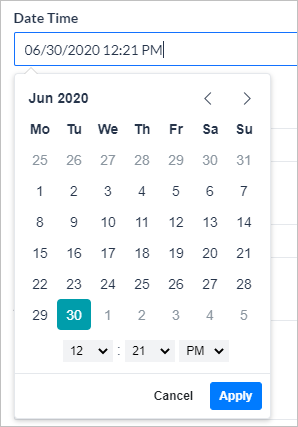The image features a white background with a light gray border forming a square along the top, left, right, and bottom edges. At the top, "Date & Time" is written in black. Below this title, there is a white rectangular shape outlined in blue, containing a text box that displays "06/30/2020 12:21 PM."

Underneath this, a smaller square menu is visible, labeled "June 2020" in black text. On the right side of this menu are arrows pointing left and right, likely used for navigation to previous and next months. Below that, the days of the week are displayed as "MO TU WE TH FR SA SU."

The calendar shows the layout of the days, indicating that June 1st is a Monday and the 30th is a Tuesday. It also includes days from the previous and following months, integrating them into the calendar view. Below the calendar, the currently selected time "12:21 PM" is displayed again, followed by two buttons: a gray "Cancel" button and a blue "Apply" button.